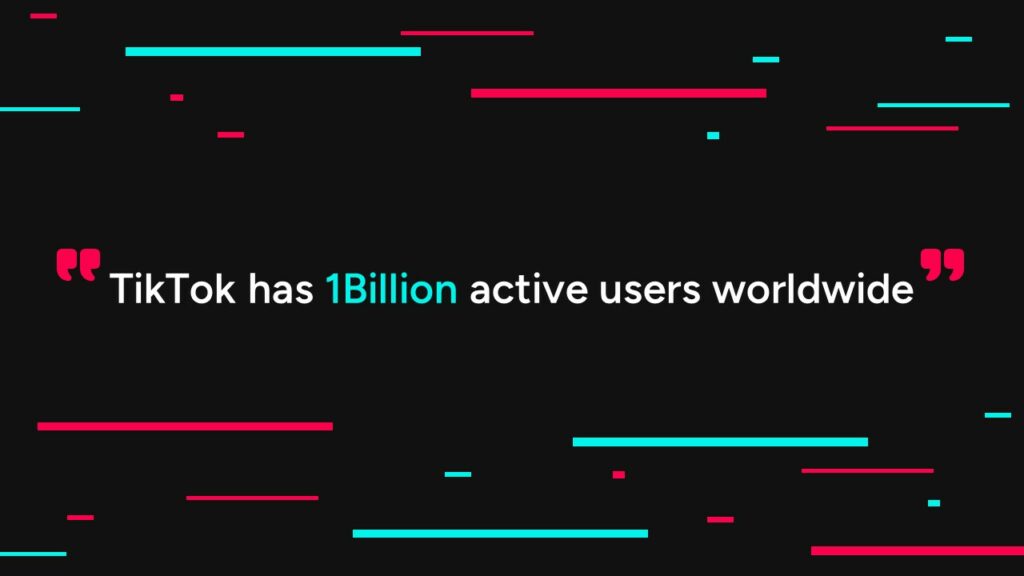In this image, we see a visually striking advertisement screenshot with a predominantly black background. Artistic lines embellish the top and bottom thirds of the frame, creating a dynamic contrast with the stark black space. These lines are rendered in two vivid colors: a bright red and a light minty green. The lengths of the lines vary, with some extending up to an inch and others no more than a dot. Their placement appears random, adding a sense of spontaneity to the design.

In the central third of the image, there is a prominent quote without any lines intersecting it, drawing the viewer's focus directly to the text. Quotation marks in bright red encase the statement, "TikTok has 1 billion active users worldwide." This quote is written in bold white print for emphasis, except for the words "1 billion," which are highlighted in the same light minty green as some of the lines, making them stand out even more in the design. The overall effect is a visually engaging and informative layout that captures attention while conveying the impressive statistic about TikTok’s user base.